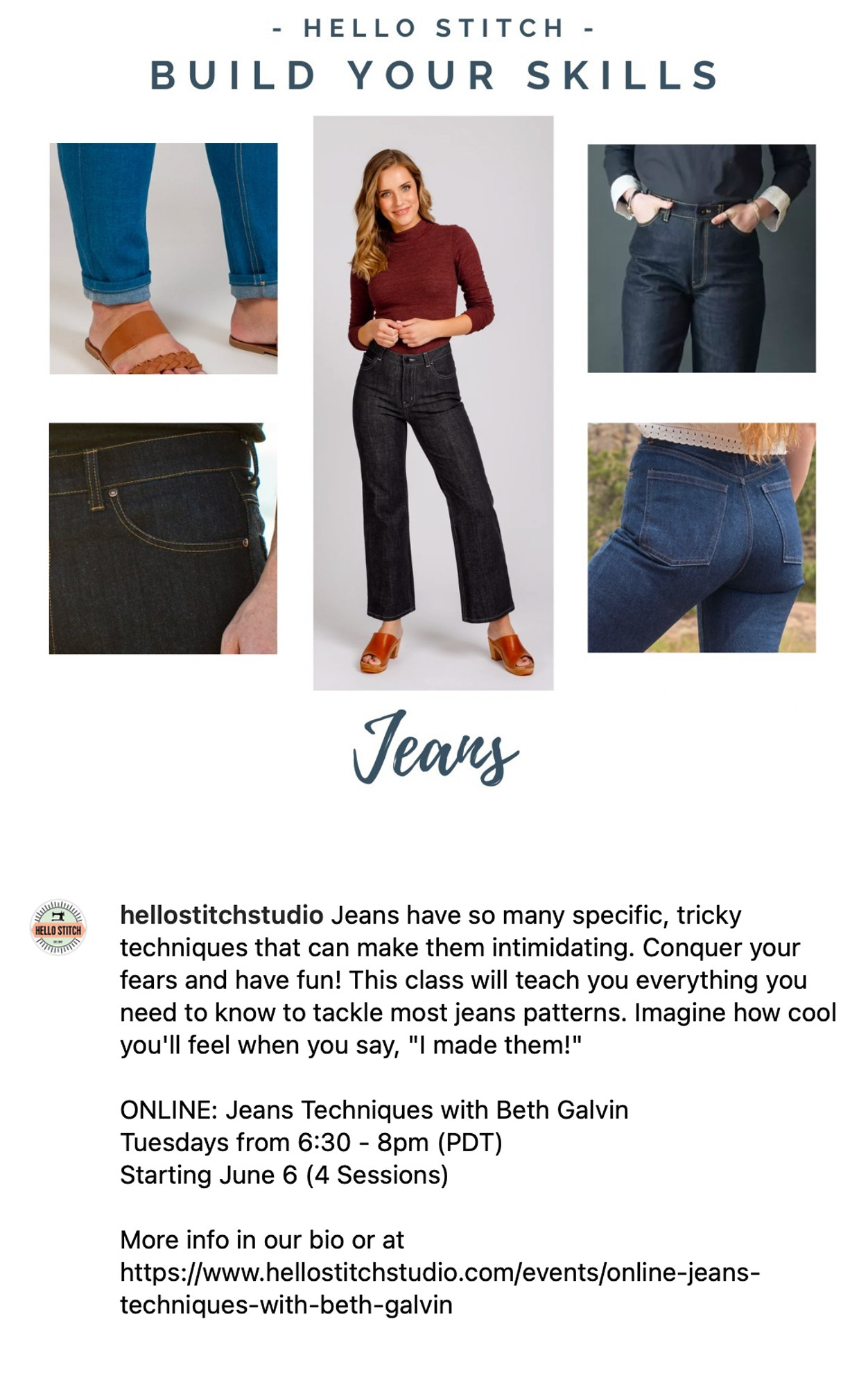This digital advertisement promotes a jeans-making class by Hello Stitch Studio. Central to the ad is a woman wearing black jeans paired with a long-sleeve burgundy shirt and sandals. Surrounding her are close-up images of jeans: the bottom of blue jeans, the pocket of black jeans, the front of jeans with hands in the pockets, and the back pockets of another pair of jeans. The ad emphasizes the message "Build Your Skills" and encourages viewers to conquer the tricky techniques of making jeans through a fun and informative class. The body text reads: "Jeans have so many specific tricky techniques that can make them intimidating. Conquer your fears and have fun. This class will teach you everything you need to know to tackle most jean patterns. Imagine how cool you'll feel when you say, 'I made them.'" The course, conducted by Beth Galvin, is titled "Online Jeans Techniques" and runs on Tuesdays from 6:30 to 8 p.m. PDT, starting June 6 for four sessions. More information can be found via their bio or at www.hellostitchstudio.com/events/online-jeans-techniques-with-Beth-Galvin.